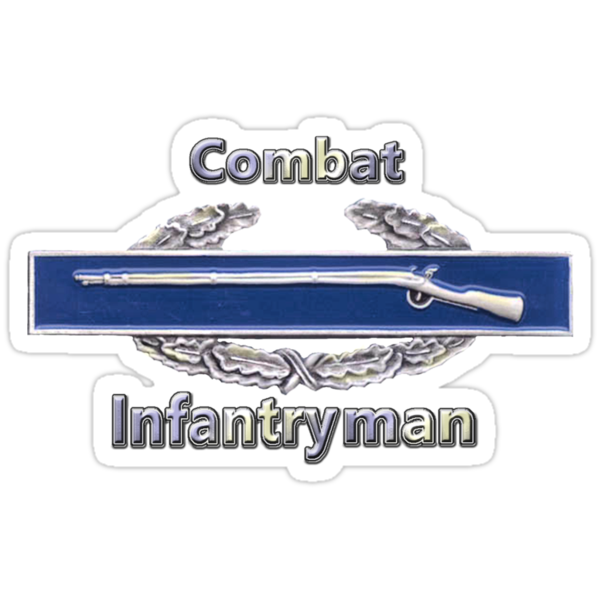The image features a distinctive white logo bordered in grey. At the top, the word "Combat" is prominently displayed, with the letters transitioning from light purple (CO) to purple and yellow (M, B) and back to purple (AT). Below this, a ring composed of greyish-green leaves encircles the central element—a bright blue box with a velvet-like texture, housing a silver, elongated rifle with its handle oriented to the right. The rifle is accentuated by the striking contrast between the blue background and its metallic sheen. Underneath the leafy ring, the word "Infantryman" appears, following the vivid color transitions similar to "Combat." The letters shift from light purple (INFA) to light yellow (NTR), back to light purple (YM), and light yellow again (AN). This visually compelling logo, which combines elements of traditional heraldry with a modern design, evokes a sense of pride, likely representing European infantry heritage.